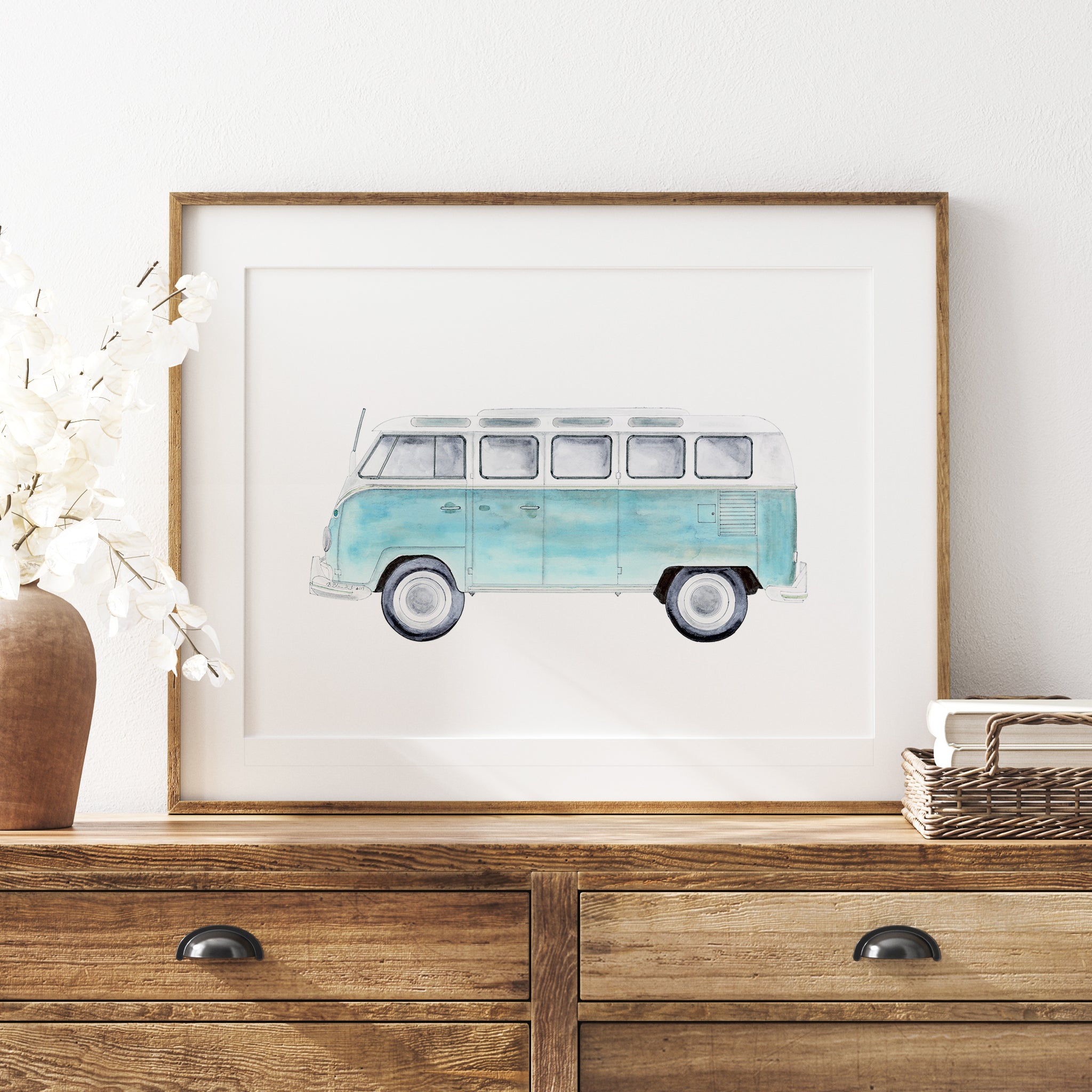In the image, a mid-to-late '60s Volkswagen bus is depicted in a simple, watercolor painting. The bus, characterized by its rounded nose, light blue lower body, and white upper section, sits prominently at the center. It features details like an antenna and distinct side windows, including four passenger windows and large driver and passenger windows, all supported by black tires with white rims. The artwork is mounted on a white mat and encased in a thin wooden frame. This framed painting rests atop a brown wooden dresser with black wooden pull handles, whose aged and unfinished wood closely matches the frame. Flanking the painting are a brown vase with white dogwood branches on the left and a wicker basket with a couple of white-bound books on the right. The scene, primarily composed of brown, black, and white tones, is rendered with a simplistic charm, with the light blue of the VW bus being the only standout color.